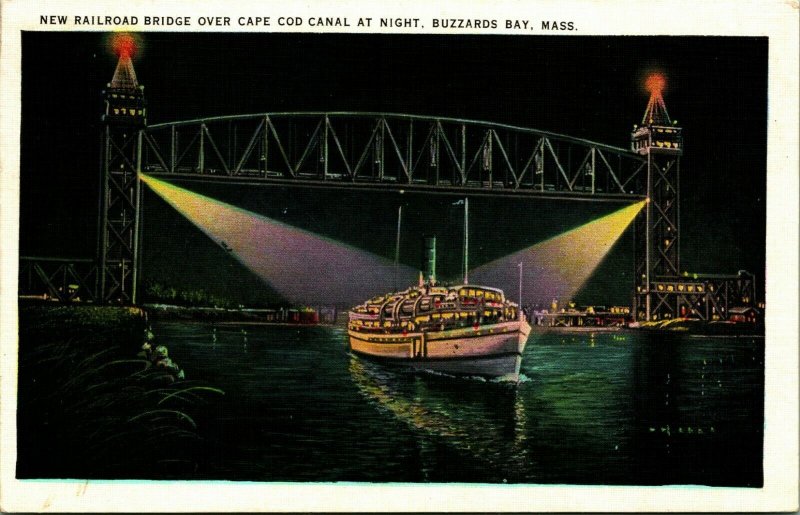This nighttime graphic artwork, presented as a postcard, depicts a white, three-deck passenger ship navigating beneath an iron railroad bridge over the Cape Cod Canal in Buzzards Bay, Massachusetts. The scene shows the ship in a 3-quarter view, heading towards the camera with its front to the right and back to the left. The bridge towers on either side rise into the dark sky, adorned with red lights at their peaks. Spotlights from these towers illuminate the ship below, reflecting off the dark water, creating visible ripples and a slight wake in front of the vessel. The postcard features a distinctive white border with the caption, "New Railroad Bridge over Cape Cod Canal at Night, Buzzards Bay, Mass." written in black at the top. The bridge, stretching across the upper middle section of the image, connects the two towers. Additional lighting details include beams shining down from where the bridge meets each tower, casting a widening glow across the ship. The ethereal lavender color and the lights around the ship’s windows add a touch of vibrancy to the midnight setting, with the body of water subtly mirroring the scene above.